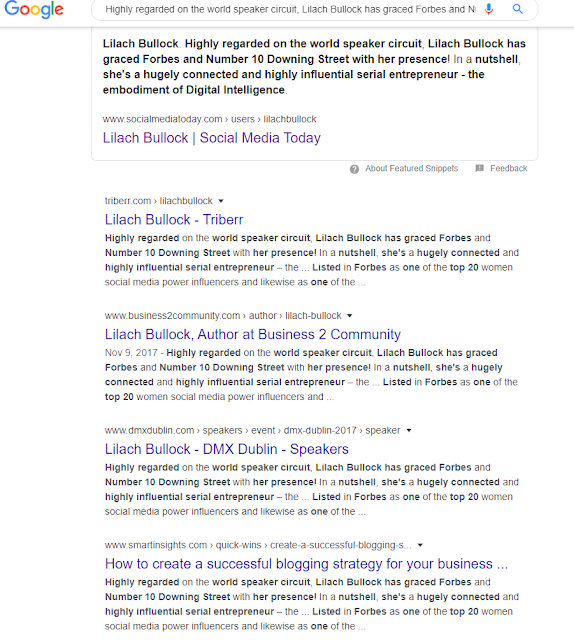The image features the iconic Google logo at the top, showcasing the brand's signature vibrant colors: blue, red, yellow, blue, green, and red. Beneath the logo, there is a search box with the highlighted text indicating that Lila Bullock is highly regarded on the world’s biggest news circuits. Lila Bullock has been praised by Forbes, indicating her prominence and influence.

The image further elaborates on her credentials by highlighting that she is "a hugely connected and highly influential senior entrepreneur," embodying digital intelligence. There are mentionings of various authoritative sources and affiliations such as:

- Social Media Today, where her name is prominently displayed in black text.
- Triber.com lists Lila Bullock twice, once in general print and again in blue text for emphasis.
- Business Community, featuring Lila Bullock as an author.
- Business2Community, highlighting her author status in blue text.
- DMX Dublin, listing her as a speaker at the 2017 event.

Consistently, the image underscores Lila Bullock's recognition across multiple platforms and dates, notably November 9th, 2017. This repetition reinforces her esteemed position and widespread acclaim in the digital and entrepreneurial community.